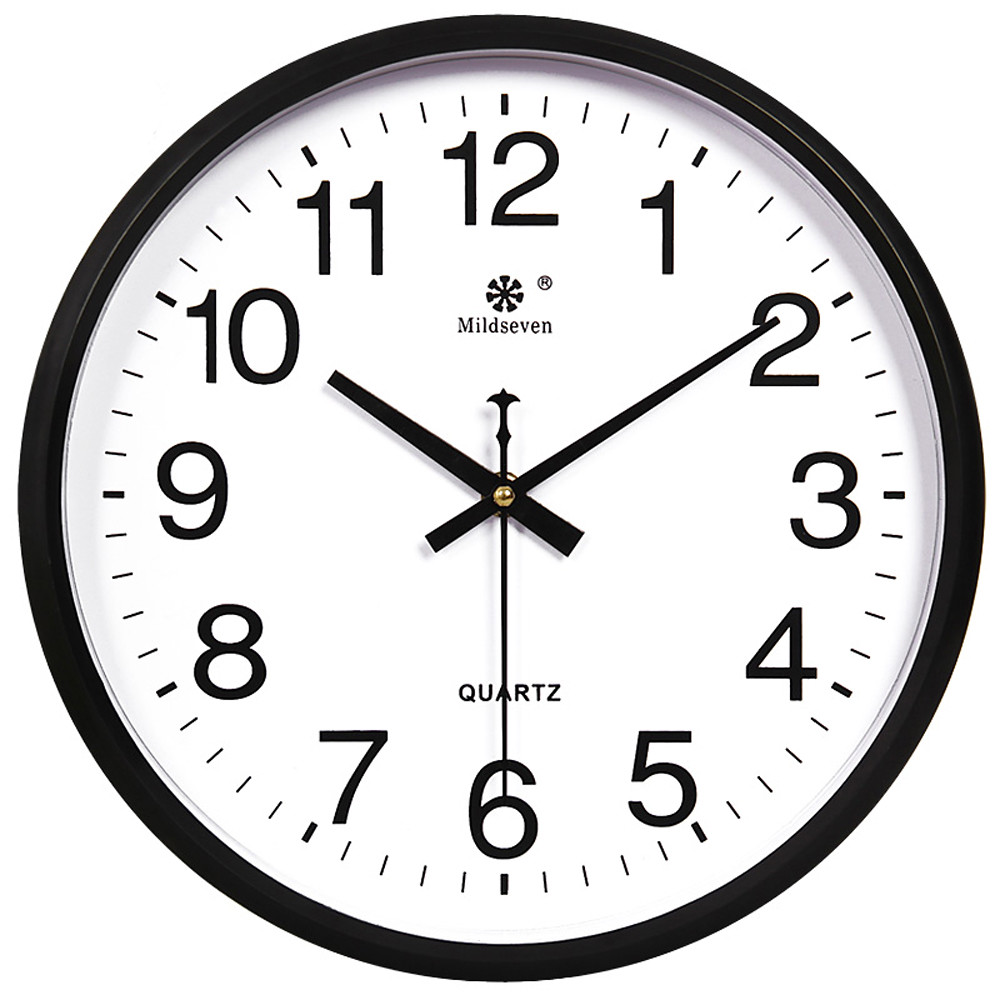The image features a round wall clock with a white face and a black plastic border. The clock prominently displays standard Arabic numerals from 1 to 12, with thinner black lines indicating each minute and darker, equally-sized lines marking the hours. At the topmost position, beneath the 12, is a logo featuring a six-pointed flower-like design, the text "Mild Seven," and a registered trademark symbol. Just above the 6, the word "Quartz" is printed in black. The clock hands are also black, with the hour hand being thicker and shorter than the longer, thinner minute hand. The thin second hand precisely points to 30 seconds. The current time shown on the clock is 10:09 and 30 seconds. The image background is plain white, making the clock's details stand out clearly.